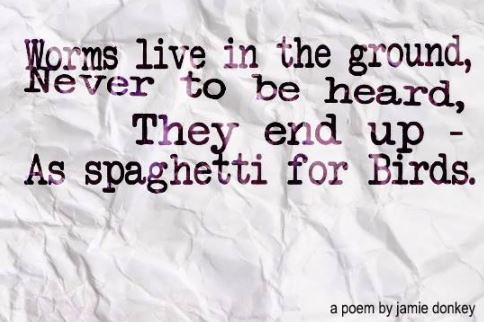On a crumpled, white, bluish-tinted piece of paper, the black text of a poem is displayed in a typewriter-style font. The text traverses the paper with a slightly uneven and diagonal alignment at the top, becoming straighter towards the bottom. The poem reads: "Worms live in the ground, never to be heard, they end up - as spaghetti for birds." Below the poem, in the bottom-right corner, the text reads: "A poem by Jamie Donkey." The entire composition creates a striking contrast with the crumpled texture of the paper against the simple, stark font.